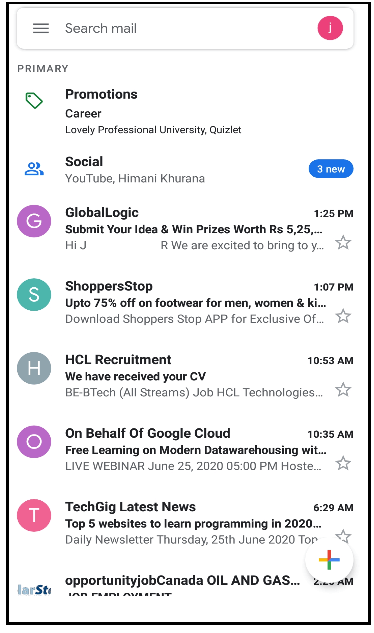The image displays a rectangular interface with a black border against a white background. At the top, there is another white rectangle with a gray outline. Inside, it says "Search email" in black text. Next to it, there are three black lines followed by a pink circle with a white "J" in the center.

Below this section, on the left-hand side, the text reads "Primary" in black. Beneath that, there are several categorized email sections:

1. **Promotions**:
   - "Career, Lovely Professional University"
   - A blue oval icon with "3 new" written in white.

2. **Social**:
   - "Global Logic Submission Idea"
   - "When prices work are 5-25-... 1:25 PM"
   - "Hi J, we are excited to bring Y..."

3. **Advertisements**:
   - "Shop with Stop: Up to 75% off on your footwear for men, women, and KI... 1:07 PM"
   - "Download Shop with Stop app for exclusive OF..."

4. **Notifications**:
   - "HCL Recruitment: We have received your CV, B.Tech or streams job at HCL Technologies... 10:53 AM"
   - "On behalf of Google Cloud: Free learning on modern data warehousing, WIT... Live webinar June 25th, 2020, 05:00 PM... host... 10:35 AM"

Each category features snippets of email content alongside respective timestamps.